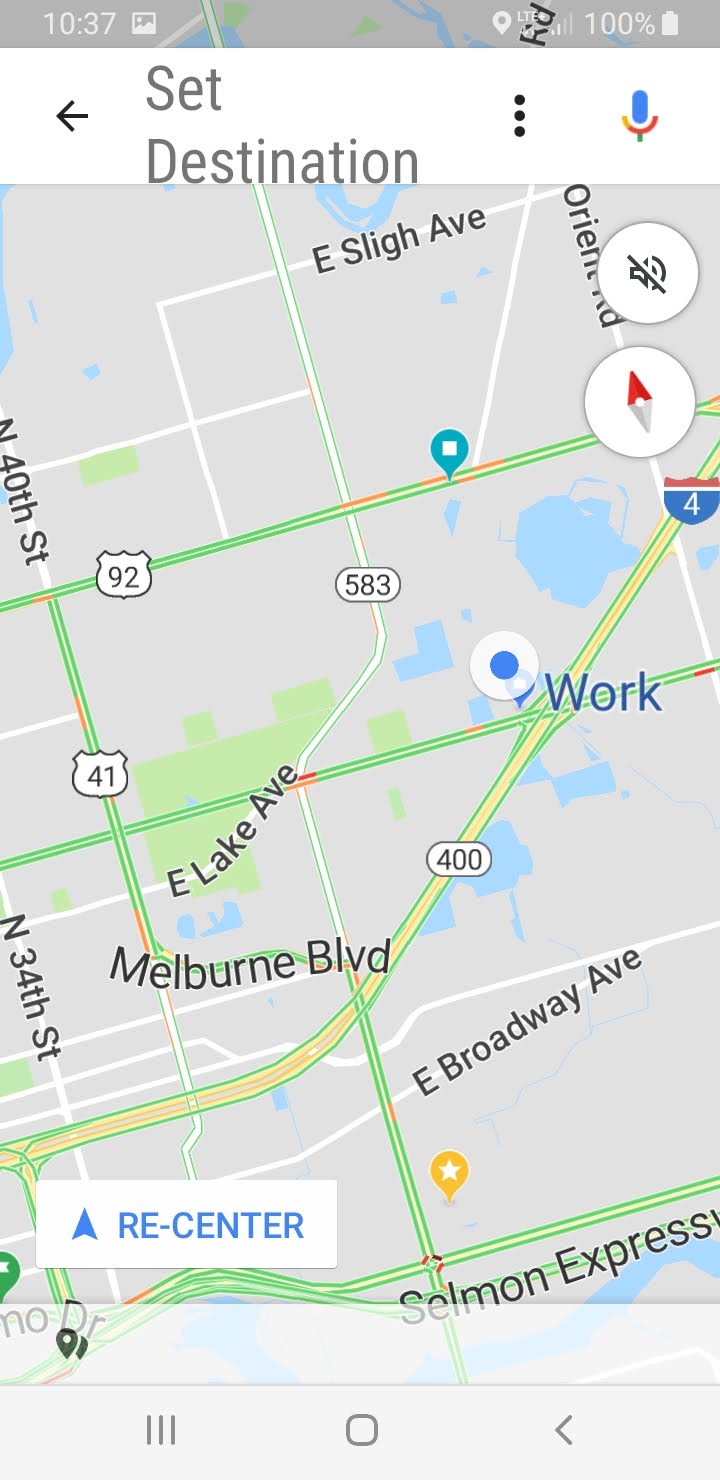The image depicts a smartphone screen showcasing a map application in use. At the top of the phone's screen, the background is gray, displaying the current time as 10:37. Within the map application, a top bar indicates "Set Destination" in gray, accompanied by a left-pointing arrow. To the right of this bar, there's a blue microphone icon followed by three vertical black dots.

On the map itself, various streets are color-coded in green, white, and yellow. A prominent blue dot with a surrounding white ring marks the location labeled "Work" in blue text. The map includes numerical indicators such as "583" and "400," each enclosed in white ovals.

A white rectangle with blue text and an upward arrow at the bottom right corner reads "Re-center." Street names are clearly visible in black text, including "East Broadway Avenue," "East Lake Avenue," "North 34th Street," and "Melbourne Boulevard." An orange location marker with a white star is also present on the map, highlighting a point of interest.